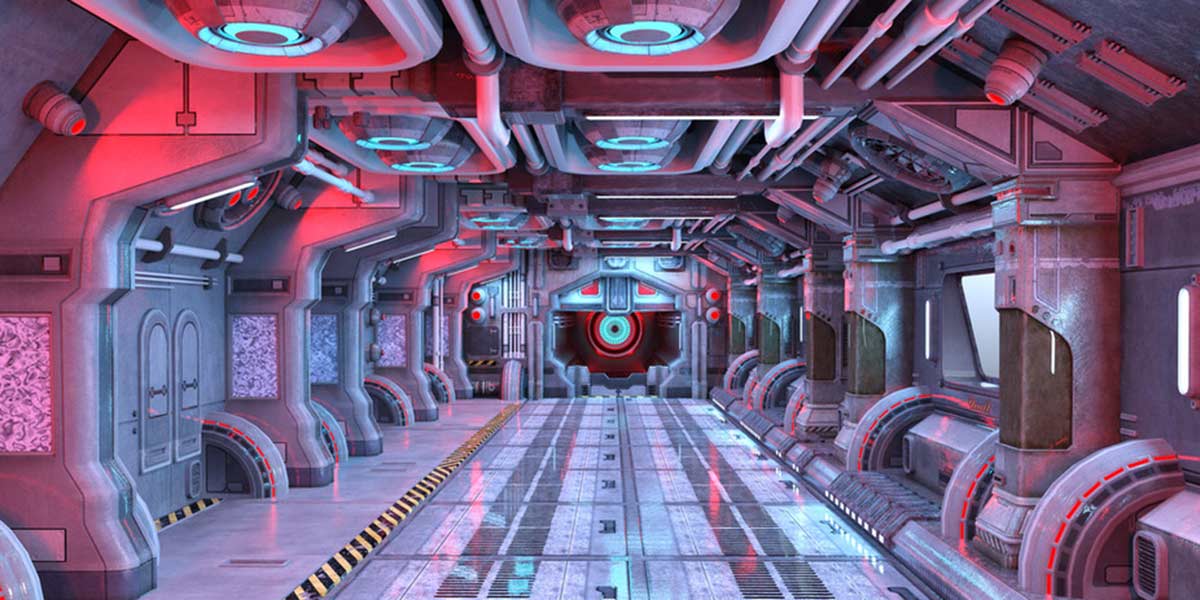The image depicts the interior of a highly futuristic, computer-generated space station or spaceship corridor. The setting is dominated by sleek, metallic gray walls and numerous structural elements that include columns rising from floor to ceiling. The corridor is lined with glowing red lights along both the walls and ceiling, enhancing the advanced and otherworldly ambiance. A prominent black and yellow caution stripe runs along the floor, contributing to the industrial aesthetic. The floor itself is shiny and reflects the myriad of lights, creating an almost luminescent pathway.

At the far end of the corridor lies a distinctive circular doorway or portal, characterized by concentric circles of red, black, and a strikingly bright light blue. In addition, the room features multiple futuristic-looking elements, including what appear to be sensors emitting red lights. Along the left side, there are either cupboards or possibly screens displaying static-like patterns, suggestive of high-tech equipment or control panels. This richly detailed scene captures the essence of an advanced spacefaring environment.